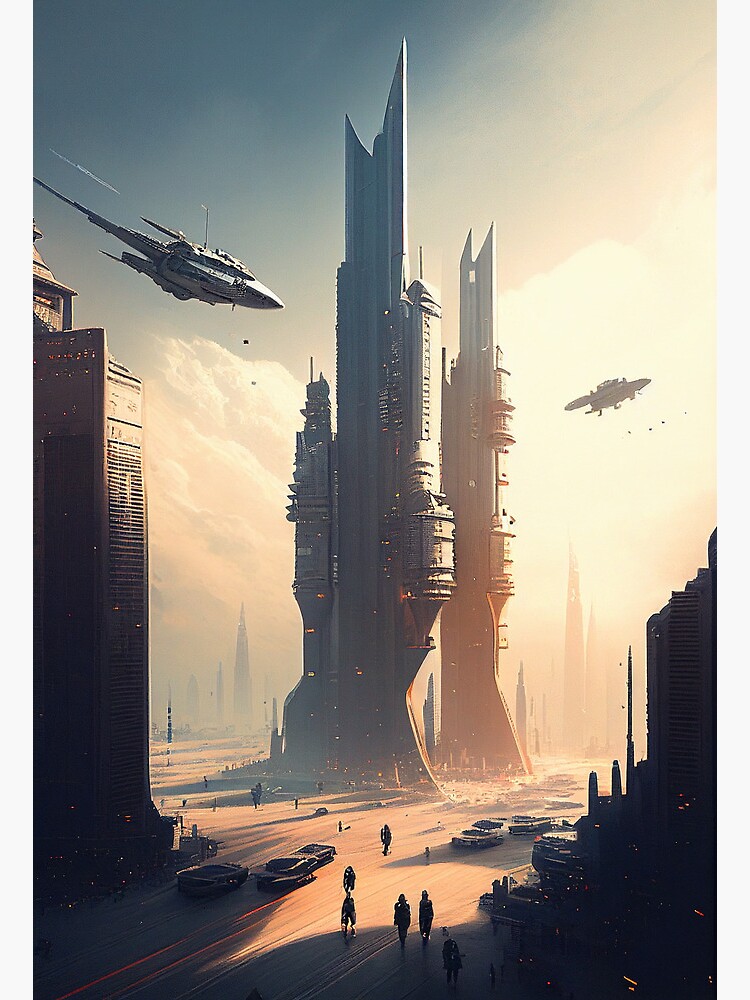The computer-generated graphic showcases a vibrant futuristic city landscape dominated by two prominent skyscrapers at its center, stylized with sharp, blade-like points that project a sense of advanced architecture. These high-rises, one resembling an upright shotgun in shape, symbolize the pinnacle of this technology-driven environment. Surrounding the central skyscrapers, various aircraft and spaceships hover and navigate at low altitudes, enhancing the city's dynamic feel. 

At ground level, the scene is bustling with pedestrians and sleek, futuristic cars, creating a lively urban atmosphere. The street level is active, with people seemingly moving towards the central hub of parked or slowly moving cars. Flanking the central high-rises are additional tall, modern buildings, partially visible and contributing to the dense skyline. 

The overall cityscape lacks greenery, emphasizing a high-tech, dried landscape under a striking blue sky adorned with clouds. A warm, orange hue, suggestive of a sunset, casts a glowing ambiance over the scene, enriching the visual depth and highlighting the contrast between the technological marvels and the natural sky.